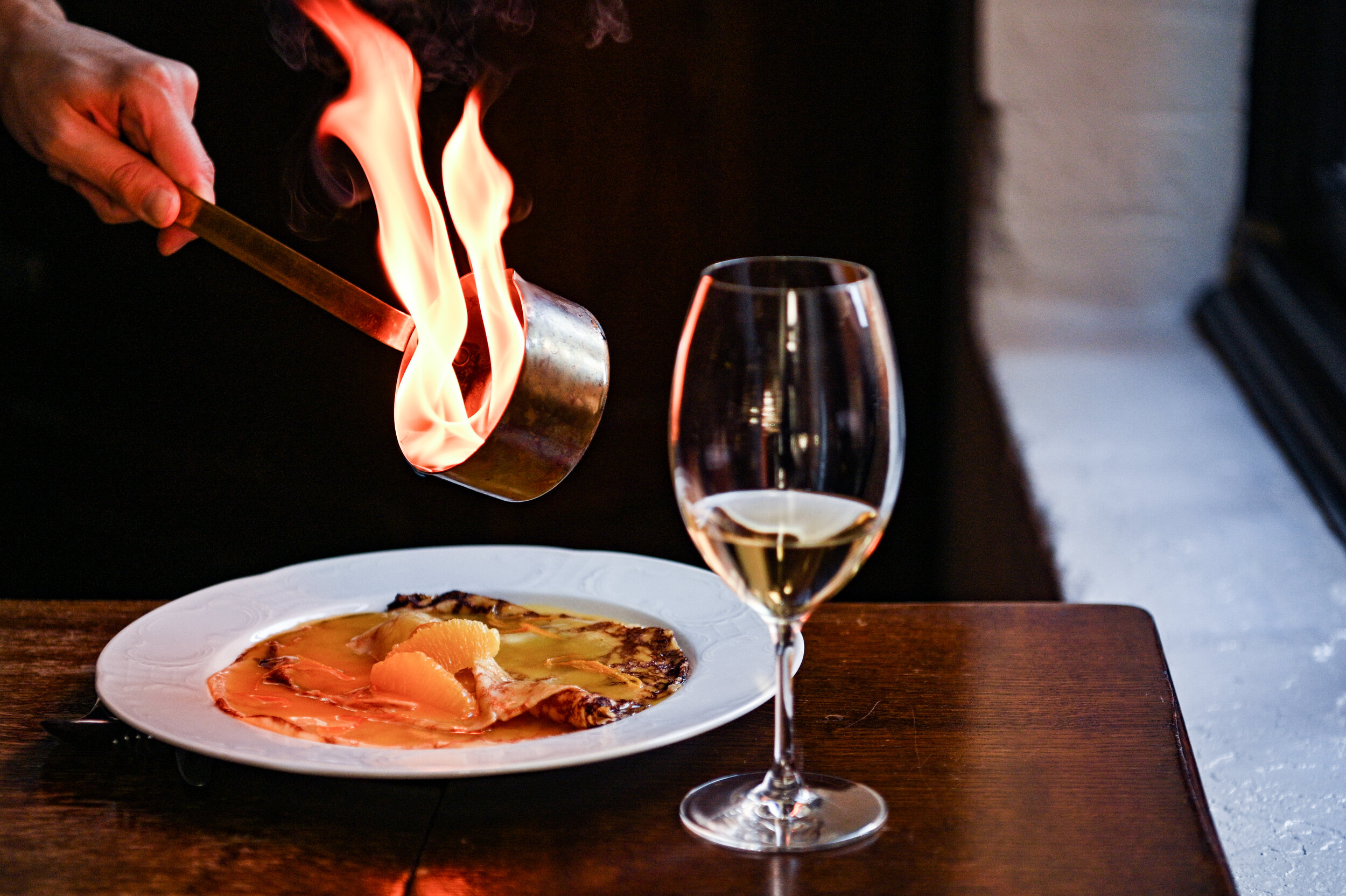This close-up image, possibly an advertisement for a restaurant or dining experience, showcases a dark brown wooden table set with a white plate containing an omelette. The omelette appears slightly overdone on the left side and burnt on the edges on the right. Just to the right and a bit forward of the plate, there is a clear wine glass about a quarter filled with white wine. Above the dish, a left hand is seen reaching into the upper left corner, holding a steel ladle filled with a flaming liquid, presumably to pour onto the dish. The background features a tall-backed dark bench and possibly a gray windowsill with a black window further to the right. The overall setting hints at a dramatic and elegant dining experience with a flambe dish as the centerpiece.